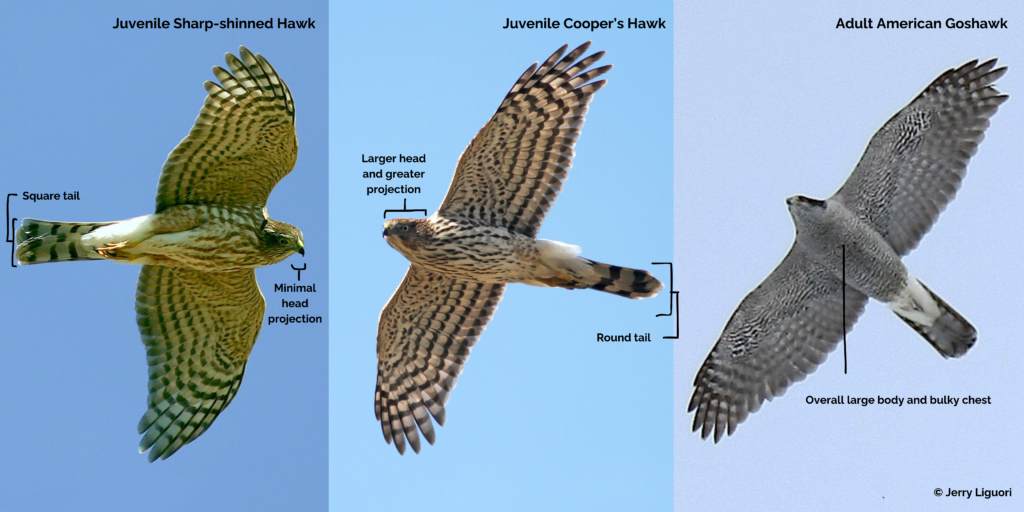This composite image showcases three different hawks in flight against a bluish-gray sky, each occupying a section of the rectangular frame. On the left, a juvenile sharp-shinned hawk is depicted, identifiable by its square tail, minimal head projection, and the distinctive underside pattern of white wings adorned with black stripes and spots, complemented by black tail bands. The middle section features a juvenile Cooper's hawk, characterized by its rounded tail and larger, more pronounced head projection; it shares a similar color scheme with black and white stripes under its wings and black body stripes. The rightmost image presents an adult American goshawk, notable for its large, robust body and bulky chest, showcasing a beautiful blend of gray, light gray, and black tones with prominent black spots and stripes. Each hawk's position and flight direction varies slightly, offering diverse views of their form and plumage. Text boxes provide informative annotations about each hawk's physical attributes, while the bottom right corner of the image credits photographer Jerry Liguori.